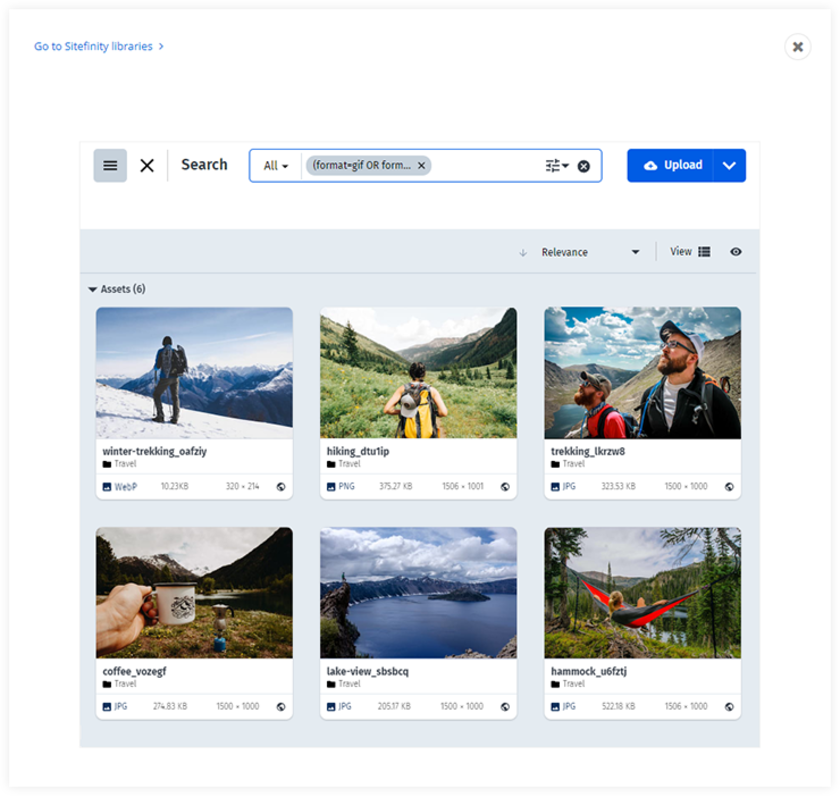The image depicts a detailed travel information webpage layout. At the top left corner, the page header features the text "Go to Sitefinity Libraries" in small blue script. Below this header, there is a search bar for users to input their travel queries. Adjacent to the search bar is a blue upload button with the word "Upload" in white text.

The main content of the page displays six vacation and adventure trip options, organized in two rows with three images each.

In the top row:
1. The first image captures a winter trekking adventure. A man, equipped with a backpack, stands on a mountaintop, gazing into the distance at a breathtaking snow-covered landscape.
2. The second image features another hiker, viewed from behind, trekking through a lush green mountain trail. The man sports a yellow backpack.
3. The third image shows two men with beards, ball caps, and glasses, looking to their left. They are outdoors in a picturesque mountainous region standing by a body of water under a clear sky.

In the bottom row:
1. The first image, labeled "Coffee," depicts a hand holding a coffee mug with a scenic mountain backdrop.
2. The second image, labeled "Lake View," showcases a stunning lake surrounded by majestic mountains and white clouds, with an island in the center of the lake.
3. The third image, labeled "Hammock," portrays an outdoor scene of a person relaxing in a hammock, though it’s difficult to determine the person’s gender. The setting appears serene with natural beauty in the background.

Each image is accompanied by labels that succinctly describe the adventure or scene depicted, providing a visually appealing overview of various travel experiences.